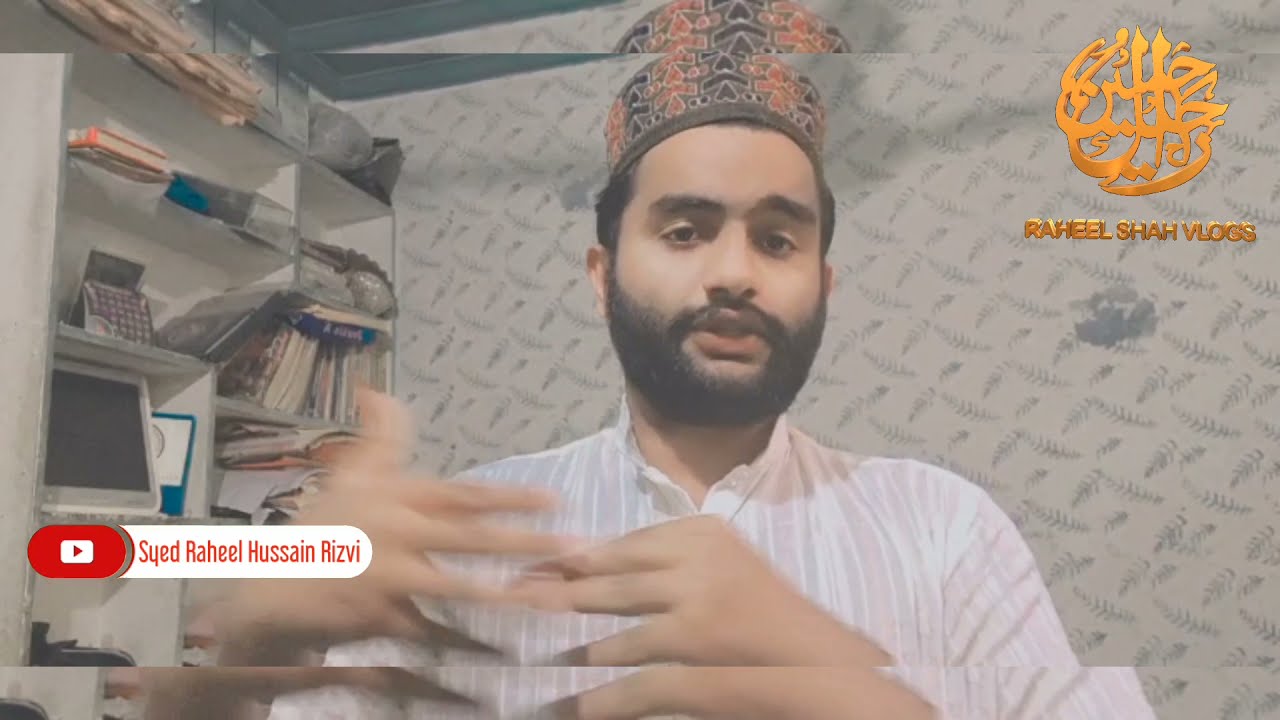The image depicts a Middle Eastern man, presumably Muslim, creating a vlog. He is captured from the chest up, wearing a white and gray striped, button-up collared shirt. He sports a dark mustache and goatee with short dark hair, and has his hands gesturing mid-motion. He wears a traditional hat with a mix of red, black, orange, and green colors. 

In the background, the office setting features a cream-colored wallpaper with a leaf pattern. To his left, there is a white bookshelf loaded with books, a computer monitor, a calculator, and some blue items, all beneath a blue ceiling. On the lower left corner of the image, there is a red YouTube play button with the name "Syed Raheel Hussain Rizvi" in red text. In the upper right corner, there's a logo in a goldish font with some Arabic script above it, reading "Raheel Shah Vlogs."